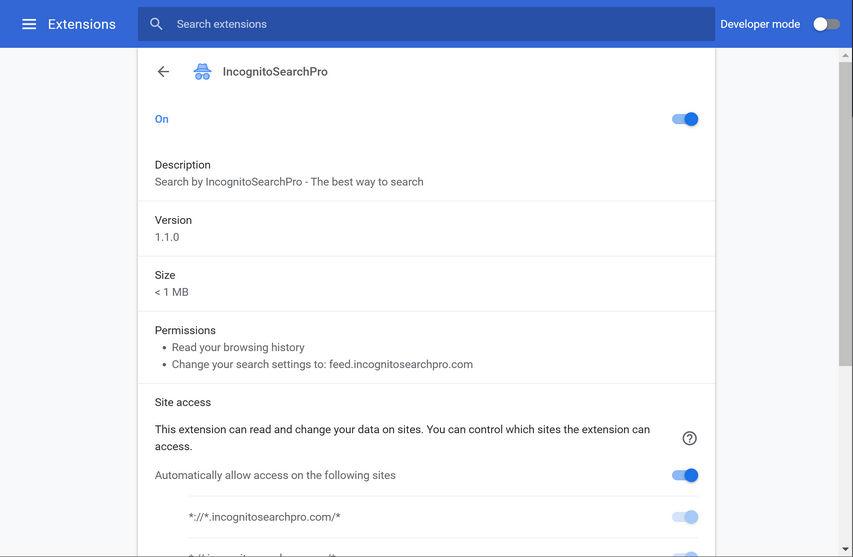Here's a detailed and cleaned-up caption for the described image:

---

This screenshot depicts the settings page of a website, characterized by its minimalistic design with dark blue text on a white background. The page is enclosed with slightly blue-shaded borders on the left and right, and a medium blue banner at the top. The top banner features "Extensions" in the upper left corner, accompanied by several clickable lines indicating options. To the right of the extensions label, there's a search bar sitting on the blue banner. In the upper right corner of the banner, there's a slider button labeled "Developer mode" in white.

Dominating the central content area of the page is information about an extension named "Incognito Search Pro," positioned in the upper left corner along with a corresponding icon. Adjacent to the name of the extension is a left arrow and an active slider button, indicating that the extension is currently enabled.

The description beneath the extension title reads, "Search by Incognito Search Pro - the best way to search." Additional details specify the version, size, and various permissions of the extension, including its ability to read and change browsing history, along with other data alterations. Site access information mentions that the extension can manage data on specified websites, with blue slider buttons available for granular control over which sites the extension can access.

Overall, the settings page presents a straightforward and user-friendly layout for managing the features and permissions of the "Incognito Search Pro" extension.